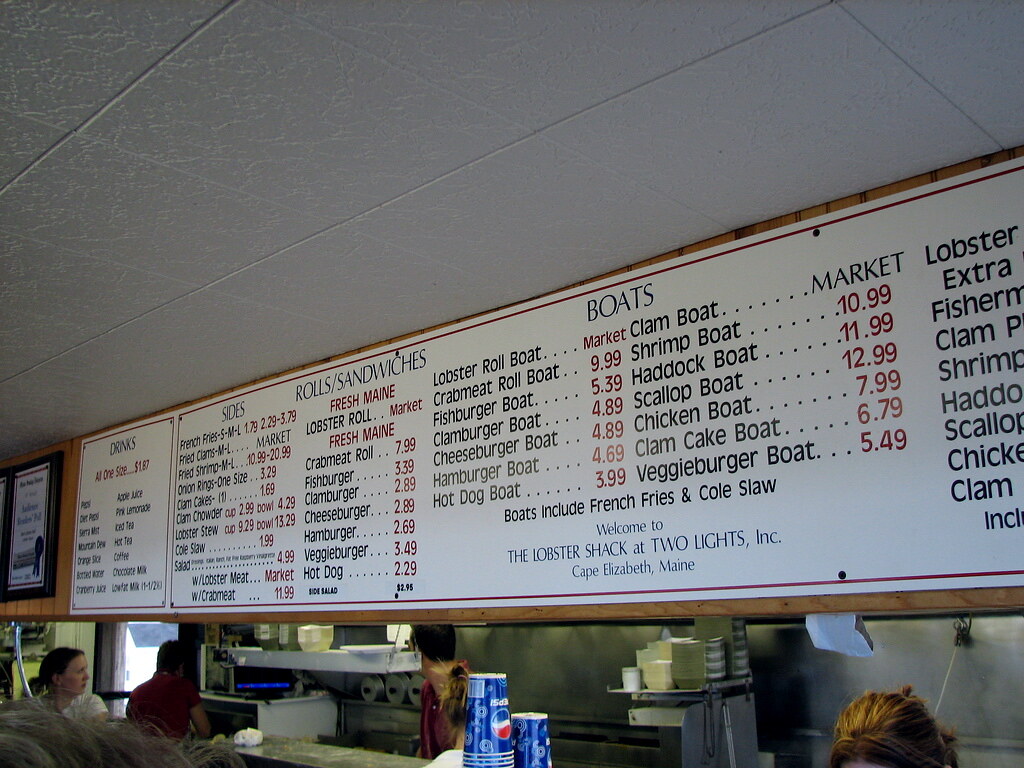This image captures a detailed view of the menu at the Lobster Shack at Two Lights, Inc., located in Cape Elizabeth, Maine. The photograph is taken indoors, featuring a white tiled ceiling at the top. The expansive menu hangs from the ceiling, dominating the central portion of the image. Directly below the menu, the kitchen area is partially visible, along with Pepsi cups, workers, and assorted kitchen tools.

The menu itself is organized into several sections on a white background. Starting from the left, the "Drinks" section lists various beverages, all priced at $1.87. The options include Pepsi, Diet Pepsi, Sierra Mist, Mountain Dew, Orange Slice, bottled water, cranberry juice, apple juice, pink lemonade, iced tea, hot tea, coffee, chocolate milk, and low-fat milk.

To the right of the drinks, the "Sides" section is displayed, offering:
- French fries in small, medium, and large sizes priced at $1.79, $2.29, and $3.79 respectively.
- Fried clams in medium and large sizes, marked as "market price."
- Fried shrimp in medium and large sizes, priced from $10.99 to $20.99.
- Onion rings (one size) for $3.29.
- Clam cakes for $1.69 each.
- Clam chowder in a cup for $2.99 or a bowl for $4.29.
- Lobster stew with a cup at $9.29 and a bowl at $13.29.
- Coleslaw at $1.99.
- Salad at $4.99 with optional dressings such as ranch and fat-free raspberry vinaigrette. There's also an option to add lobster meat (market price) or crab meat for $11.99.

Next, the "Rolls/Sandwiches" section includes:
- Fresh Maine lobster roll at market price.
- Fresh Maine crab meat roll for $7.99.
- Fish burger at $3.39.
- Clam burger for $2.89.
- Cheeseburger at $2.89.
- Hamburger for $2.69.
- Veggie burger at $3.49.
- Hot dog for $2.29.

Further to the right, the "Boats" section features meal combinations, which include french fries and coleslaw, with the following options:
- Lobster roll boat at market price.
- Crab meat roll boat for $9.99.
- Fish burger boat at $5.39.
- Clam burger boat for $4.89.
- Cheeseburger boat for $4.89.
- Hamburger boat at $4.69.
- Hot dog boat for $3.99.
- Clam boat at market price.
- Shrimp boat for $10.99.
- Haddock boat is $11.99.
- Scallop boat for $12.99.
- Chicken boat at $7.99.
- Clam cake boat for $6.79.
- Veggie burger boat at $5.49.

The menu continues beyond the right edge of the frame, indicating additional offerings not visible in this image. The entire setup emphasizes the diverse offerings of this reputed seafood restaurant, providing a clear and accessible overview of its food and drink selections.